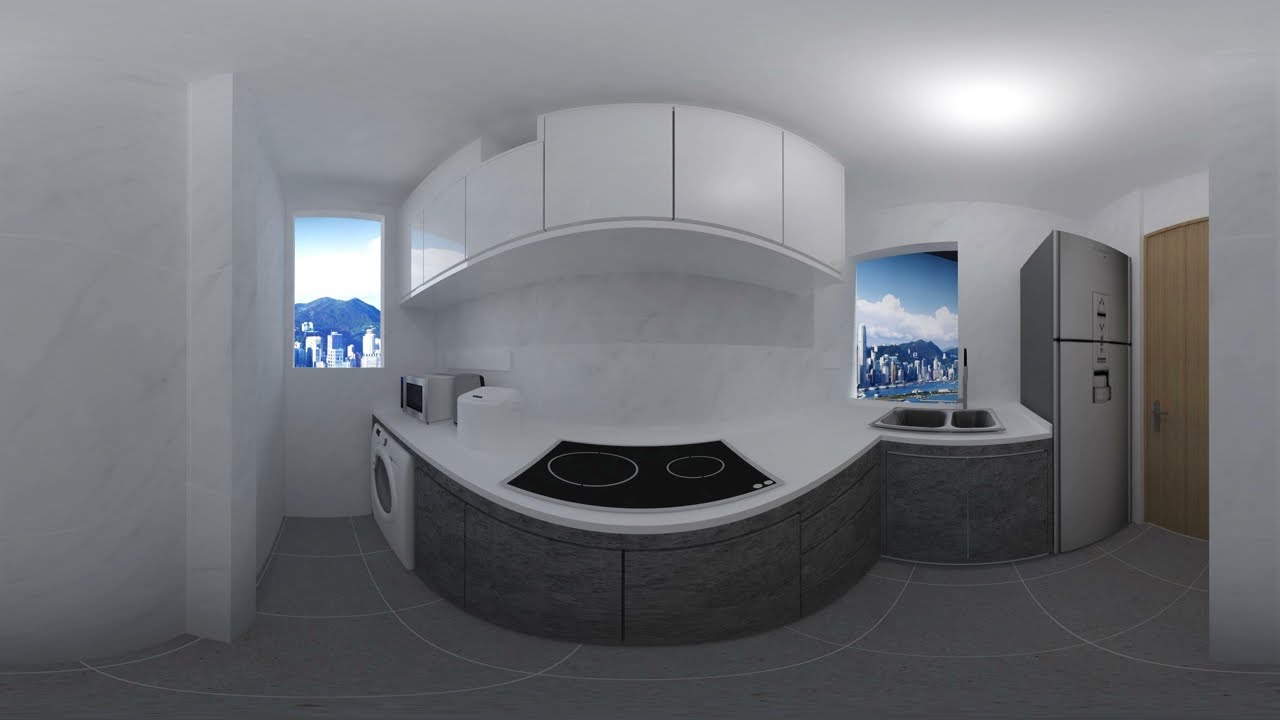This photograph showcases a modern, panoramic view of a kitchen with a sleek, contemporary design. The center of the kitchen features a blue induction cooktop with white circular designs, set into an oval-shaped white countertop. Above the cooktop, curving along the edge of the counter, are white cabinetry. Flanking the cooktop on both sides are two large windows that provide a scenic view of the cityscape, hills, and sky.

To the left of the cooktop, there is a knee-high washing machine and a counter that holds a microwave and a white electric pot. Below this counter are grey cabinets, while additional white cabinets are mounted on the wall above. On the far left stands a grey refrigerator, adjacent to the brown wooden kitchen door.

To the right of the cooktop and near the corner of the kitchen, there is a double-bay kitchen sink set into the counter. The kitchen is visually unified with white walls, a white ceiling, a grey tiled floor, and modern appliances that enhance its sleek aesthetic.